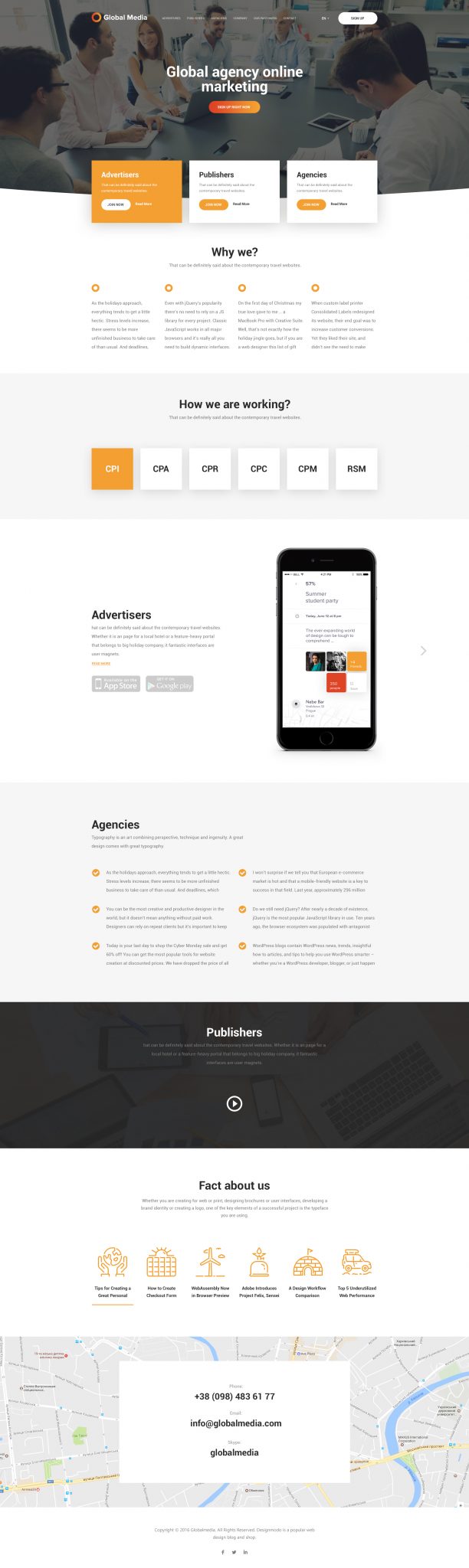Here is a refined and detailed caption for the image:

"The screenshot displays a comprehensive landing page for a global online agency. At the top, the header reads 'Global Agency Online,' providing a panoramic view of the entire page. Central elements include three distinct buttons: one orange square with a white button and two white squares with orange buttons, followed by a section titled 'Why We?' with four paragraphs of explanatory text in small, nearly unreadable font. Beneath this, there are six clickable boxes that turn orange when selected, leading into sections titled 'How Are We Working?' and 'Agencies & Publishing.' Additionally, the page contains a segment labeled 'Facts About Us,' featuring small icons to illustrate the information provided. Towards the bottom, a map showcases the agency's location, accompanied by contact details such as a phone number and email address. The page concludes with social media icons for further engagement."